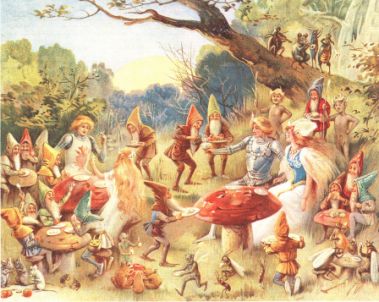In the image, we're looking at a detailed painting that portrays a lively garden party scene with a medieval, fairy-tale theme. The setting is a sunny grass field, just on the edge of a forest, filled with vibrant colors—reds, light oranges, browns, greens, beige, tan, whites, blacks, and grays. 

Foreground elements include large mushrooms serving as table tops around which several small, gnome-like dwarves with long white beards and colorful pointy hats are gathered. Many have plates in their hands, suggesting they are partaking in a meal or celebration. Scattered amongst the gnomes are four human-sized figures dressed in medieval attire, with the men appearing to wear armor. On the left, there is a blonde-haired man and a woman with long blonde hair. On the right, another pair consists of a man with ginger-blondish hair and a woman with long ginger hair. 

A tree extends from the top-middle of the painting, arching towards the right side, adding depth to the scene. In the background, there are additional trees hinting at the forest beyond. The overall atmosphere is cheerful and festive, with both the dwarves and humans displaying positive facial expressions, suggesting they're enjoying a joyful event.